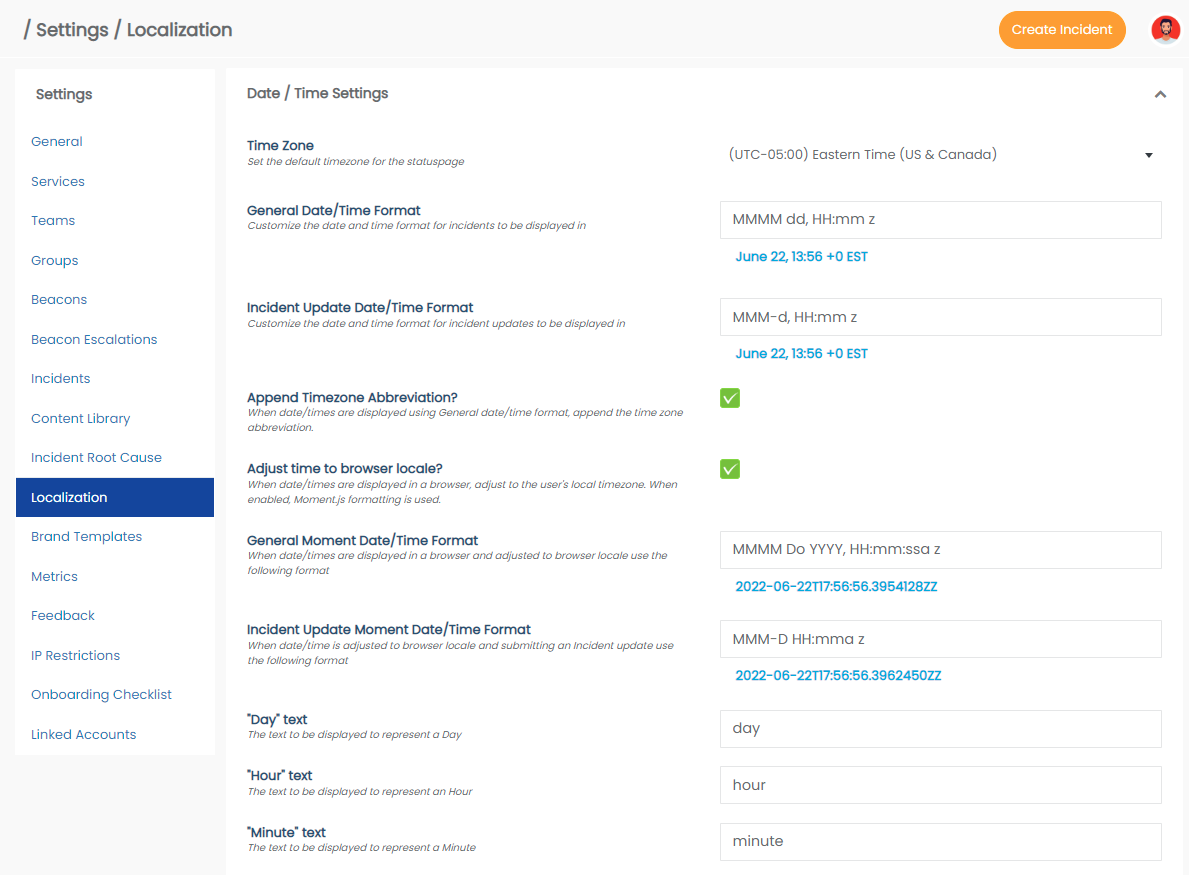In this image, we are viewing a screenshot of a user interface. Starting from the top, there is a light gray header. In the upper-left corner of the header, the word "Settings" is displayed in black text. To the upper-right, there is an orange action button labeled "Create Incident."

Below the header, in the center, there is a caricature image of a young man enclosed in a red circle. 

On the left side of the screenshot, there is a vertical white navigation menu. The menu is titled "Settings" in bold black text at the top. Underneath "Settings," in gray text, there are various menu items listed: "General," "Services," "Teams," "Groups," "Beacons," "Beacon Escalations," "Incidents," "Content Library," "Incident Root Cause," and a highlighted item in a dark blue box labeled "Localization." Further down, additional menu items include "Brand Templates," "Metrics," "Feedback," "IP Restrictions," and "Onboarding Checklist."